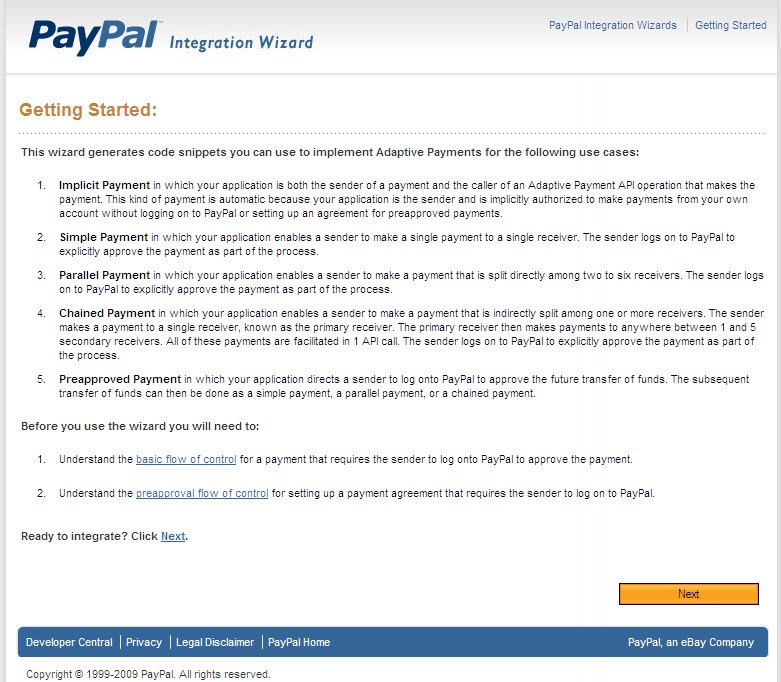Here is a detailed and cleaned-up caption for the image based on your description:

---

The screenshot displays the PayPal Integration Wizard interface, accompanied by various navigation and instructional elements. At the top, the PayPal logo is prominently featured, showcasing the brand name in dark and light blue. Adjacent to the logo, the title "Integration Wizard" is presented in a smaller font. 

Below the logo, the section titled "Getting Started" is highlighted in orange, followed by a set of instructions designed to guide users through the initial steps of using the wizard. The instructions clarify that the wizard generates code snippets for several payment scenarios, including implicit payments, simple payments, parallel payments, chain payments, and pre-approved payments.

Before proceeding, users are advised to understand two key concepts: the basic flow of control for a payment, which includes logging onto PayPal to approve the payment, and the pre-approval flow of control for setting up a payment agreement. Both "basic flow of control" and "pre-approval flow of control" are hyperlinked, underlined, and colored blue to indicate clickable links for further information.

At the bottom of the page, users are prompted with the question "Ready to integrate?" followed by a clickable hyperlink labeled "Next." In addition to this textual link, a prominent orange rectangular button with the word "Next" in black is located near the bottom right, providing an alternative way to proceed with the integration process.

The footer of the interface features a narrow blue bar that includes various options such as Developer Central, Privacy, Legal Disclaimer, and PayPal Home. It is also noted that PayPal is an eBay company, which is stated next to the navigation options.

---

This caption provides a comprehensive and organized description of the PayPal Integration Wizard interface, highlighting key elements and navigational aids present in the screenshot.